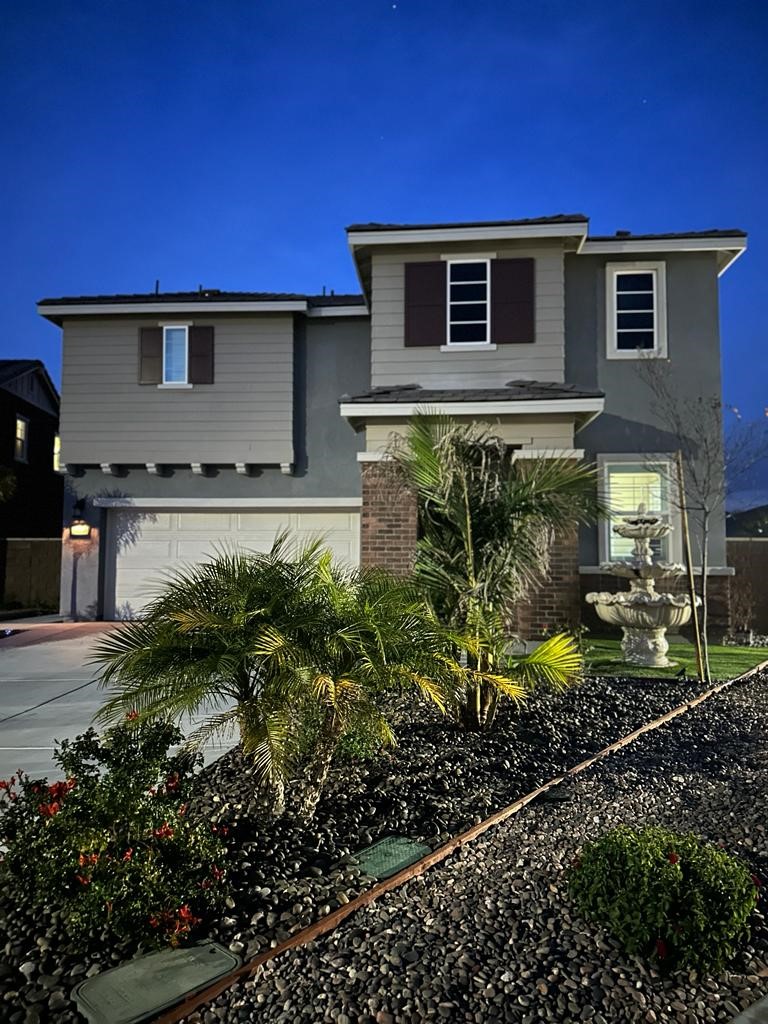The photograph captures a detailed front view of a two-story contemporary house, taken from the sidewalk or street. The house exudes a wealthier aesthetic with its intricate design elements. The exterior boasts a mix of gray stucco and gray siding, adorned with black shutters and white trim. On the left, there's a prominent two-door white garage, over which sits a small room with a tiny window framed by black shutters. The house features two brick pillars that frame the obscured front door, partially hidden by a lush, flowering bush and a mini palm tree or large fern. Further right, the lower part of the house is bordered with brick, while the upper part continues the gray stucco theme, punctuated by two windows. The well-maintained front yard showcases a blend of greenery, including several types of bushes and small trees. The ground is primarily covered in pebbles with a patch of green grass in the middle, home to a striking three-level, white ceramic water fountain. A concrete driveway snakes up to the garage, and a black light fixture near the garage is illuminated, casting a warm yellow glow, indicating the onset of dusk.